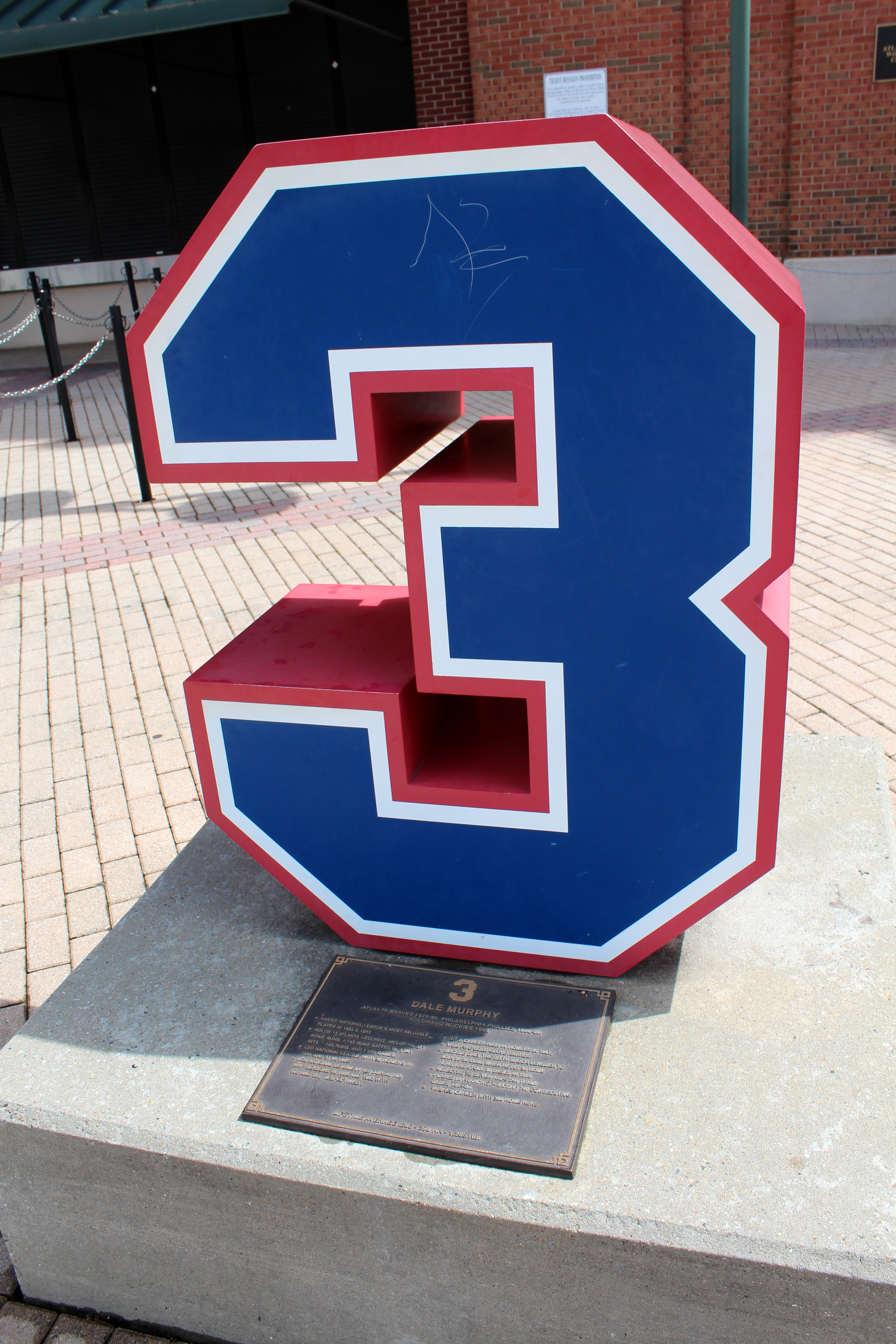The image depicts an outdoor daytime setting, likely outside a baseball stadium. Central to the image is a large cement statue of the number three. The statue is prominently blue with white inner borders and a red outline. At the top of the blue section, there is a marking that could be a signature, graffiti, or simply a scuff.

The base of the statue features a dark brown plaque with gold trim, displaying the number 3 and the name Dale Murphy, a renowned baseball player, in gold lettering. Below his name, there are two small paragraphs of text, aligned to the left and right, though they are too small to read clearly.

The ground surrounding the statue is covered in light cream to light brown brick-style flooring. In the bottom right corner of the image, there is a stone slab with the number 3 and some unreadable text beneath it. In the background, there is a red brick building partly visible at the top of the image, along with green and black poles connected by a silver chain, likely used for crowd control. The presence of the Sun casting shadows indicates that the photo was taken in daylight.